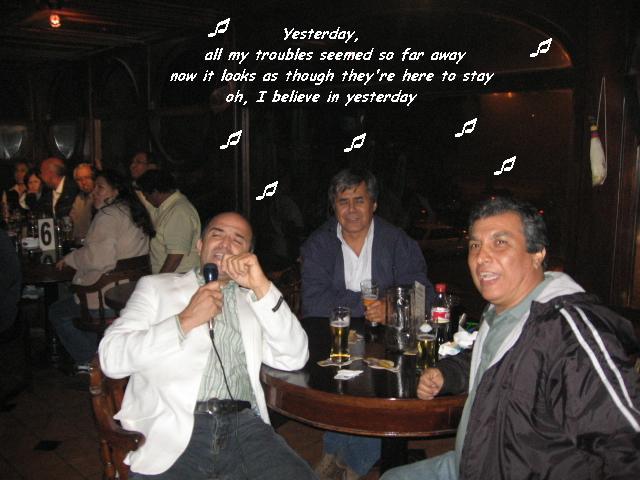This photograph captures a lively karaoke session set in a dimly lit bar with a warm, cozy ambiance. At the forefront, three men, possibly of Hispanic or Middle Eastern descent, are seated around a dark wooden round table adorned with glasses filled with beer, a plastic Coca-Cola bottle, and some napkins. The man on the left, distinguished by his white jacket, black jeans, and pinstripe shirt, holds a microphone and is evidently singing passionately with his eyes closed and one hand raised to his mouth. At the center of the trio sits a man with gray hair, clad in a dark jacket and a white button-up shirt, also seemingly engrossed in the song with his eyes shut. To the far right, the third man wears a black windbreaker, a green shirt, and jeans, and his open mouth suggests he is singing along as well.

In the background, a mixed group of men and women, predominantly Caucasian, can be seen gathered around a table marked with the number six, adding to the bustling, communal atmosphere of the scene. Above, white musical notes frame the lyrics, "Yesterday, all my troubles seemed so far away, now it looks as though they're here to stay. Oh, I believe in yesterday," emphasizing the nostalgic tone of the moment being shared.